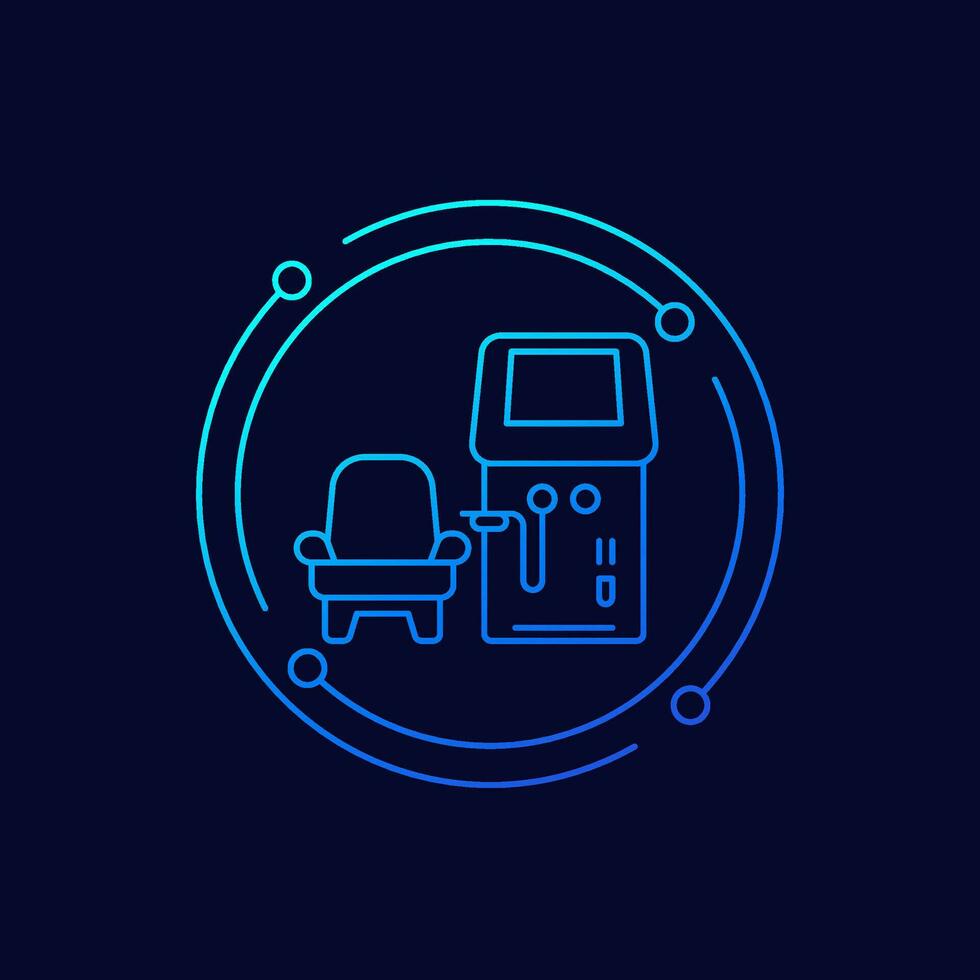The image features a dark blue background with a circular logo in the center that gradients from a light blue on top to a darker blue at the bottom. Within this circle, there is minimalistic artwork outlined in neon bluish-green hues. On the right side of the circle, there is a rudimentary drawing of a gas pump, characterized by a square screen with another smaller square inside it, situated at the top of the pump. Below the screen are two small circles and a line resembling a hose that extends downward. Additionally, there are two slots on the right side of the gas pump. To the left of this gas pump is an outline of a living room armchair, simple yet distinct in its minimalist style. The overall composition of the logo gives a sleek and modern aesthetic, with a hint of vintage charm due to the gas pump and armchair elements.